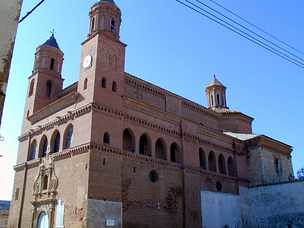This is an image showing the exterior of an old, brick building resembling a church, characterized by its classic architecture. The building is primarily a light brown or brownish-red hue and features multiple towers with pointed roofs, one of which has a visible cross. Arched windows adorn the front and side sections, with four arched windows notable on what appears to be the third story. The front façade includes a large clock and two prominent columns rising to peaks. The left side of the image reveals a white door. The sky above is clear and blue, and a few electrical wires are visible at the top. Although the image is somewhat blurry, these distinct architectural elements stand out clearly.